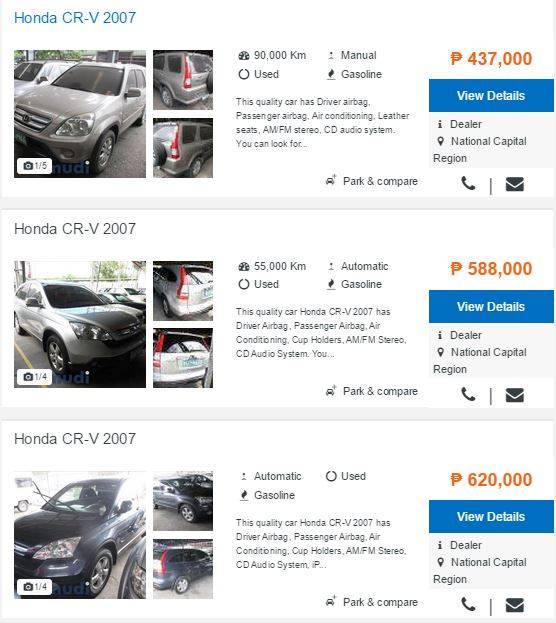The image displays a comparison of three Honda CR-V 2007 models available for sale.

### Top Left Section:
#### Car 1:
- **Model:** Honda CR-V 2007 (Blue)
- **Color:** Silver Grey
- **Mileage:** 90,000 kilometers
- **Transmission:** Manual
- **Fuel Type:** Gasoline
- **Features:** Driver airbag, passenger airbag, air conditioning, leather seats, AM/FM stereo, and a CD audio system.
- **Price:** ₱437,000 (in orange text)
- **Additional Options:** "View Details" button (blue), "Park and Compare," "Call," and "Email" buttons.
- **Location:** iDealer, National Capital Region

### Second Section:
#### Car 2:
- **Model:** Honda CR-V 2007 (Silver Grey)
- **Color:** Silver Grey
- **Mileage:** 55,000 kilometers
- **Transmission:** Automatic
- **Fuel Type:** Gasoline
- **Features:** Driver airbag, passenger airbag, air conditioning, cup holders, AM/FM stereo audio system.
- **Price:** ₱788,000 (in orange text)
- **Additional Options:** "View Details" button (blue), "Park and Compare," "Call," and "Email" buttons.
- **Location:** iDealer, National Capital Region

### Third Section:
#### Car 3:
- **Model:** Honda CR-V 2007 (Dark Blue)
- **Color:** Slightly Dark Blue
- **Mileage:** Not specified
- **Transmission:** Automatic
- **Fuel Type:** Gasoline
- **Features:** Not specified in detail but implied to have basic Honda CR-V 2007 features.
- **Price:** ₱620,000 (in orange text)
- **Additional Options:** "View Details" button (blue), "Park and Compare," "Call," and "Email" buttons.
- **Location:** iDealer, National Capital Region